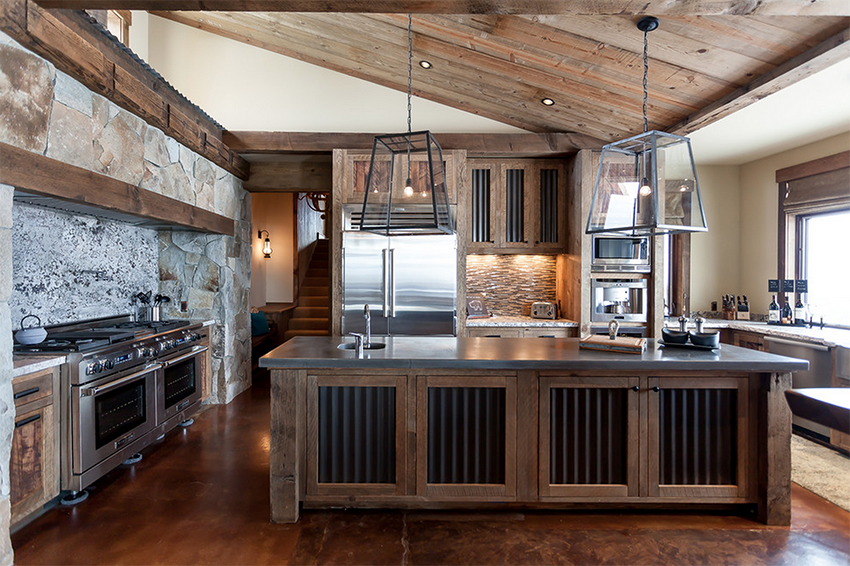This photo showcases a beautifully designed kitchen with a rustic industrial style. The ceiling features dark-stained wooden slats accented with small round lights and two prominent hanging fixtures. These fixtures consist of bare Edison bulbs encased in glass-paneled cages rimmed with black metal. A large island, constructed with dark wood cabinets that have black curtains, dominates the center of the kitchen. Atop the island is a dark marble countertop with two integrated sinks. Along the left wall, which is adorned with stone, stand two identical stainless steel stoves with matching ovens. A kettle sits atop one of the stoves. A flight of stairs is visible through a doorway on this side, ascending from the kitchen floor, which is also a dark hardwood. In the middle of the image, there is a striking, silver reflective refrigerator. To the right, additional wooden cabinetry is complemented by a countertop that holds a toaster and displays several liquor and wine bottles. A large window on this side allows natural light to fill the room, with a counter situated just below it. Overall, the kitchen exudes a cohesive blend of industrial elements and rustic charm.